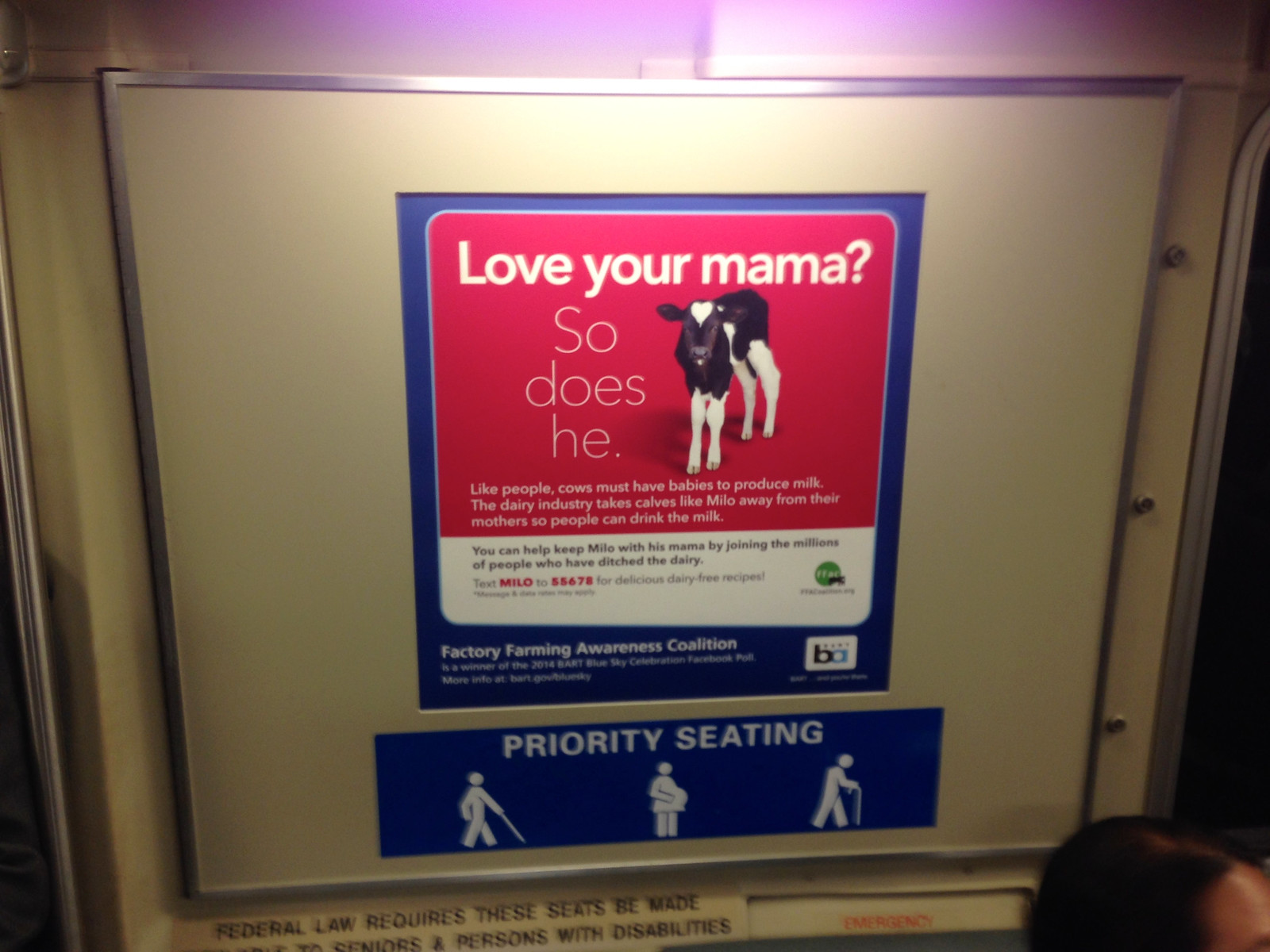This image captures an advertisement and priority seating sign inside a public transportation vehicle, likely a bus, train, or subway. The primary focus is an impactful poster from the Factory Farming Awareness Coalition placed above the seats. The poster features a blue border with a red background and white text that reads, "Love your mama, so does he," accompanied by a photo of a cow. The text explains that, like humans, cows need to have babies to produce milk and highlights the practice of separating calves like Milo from their mothers in the dairy industry for milk production. It encourages people to help keep milk with the calves’ mothers by ditching dairy, providing ways to text for more information. Below this advertisement, there is a blue rectangular sign indicating "Priority Seating" with white icons representing a person with a cane, a pregnant woman, and a blind person with a walking stick, alongside other regulatory information about seating accommodations for seniors and persons with disabilities. This signage is mounted on a partition or panel above the seating area in an indoor transit setting.